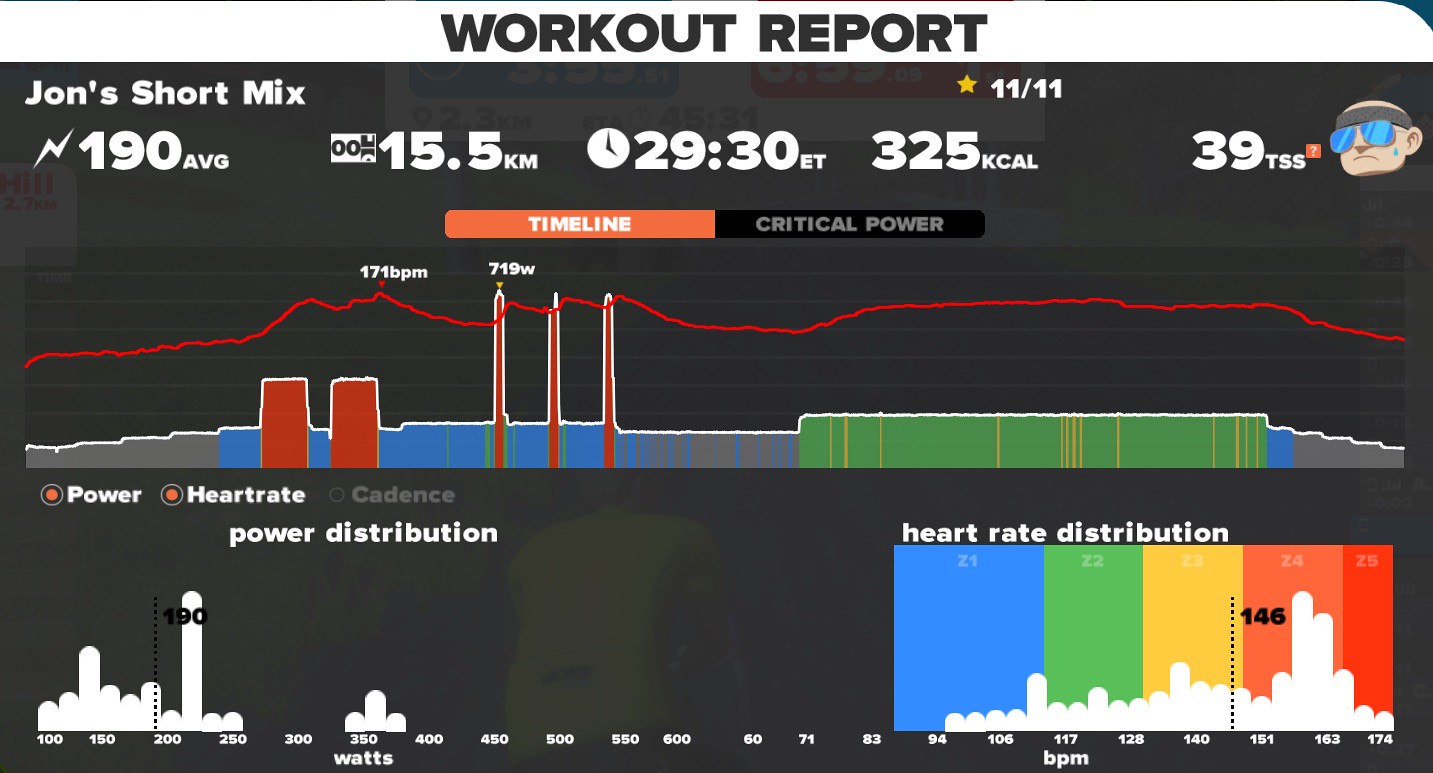The image appears to be a cropped screenshot displaying a detailed "Workout Report" for John's short mix. The top section features a white band with a dark font title. Visible statistics include a white lightning bolt icon followed by "190 average," "15.5 kilometers," "2930 time," "325 kilocalories," and "3339 TSS." Below these stats, two buttons labeled "Timeline" and "Critical Power" are shown, with "Timeline" being highlighted. The main section of the image depicts a fluctuating graph with a curve that rises and falls over time. The lower portion of the graph includes various colored sections, indicating measurements of different metrics.